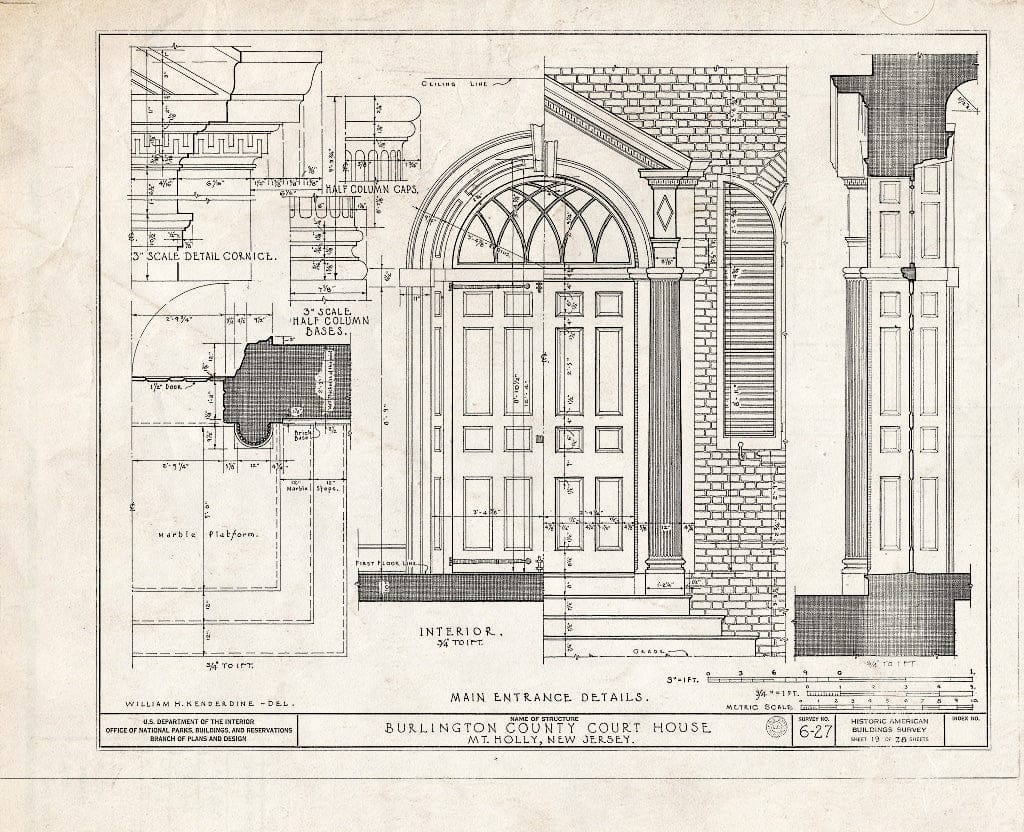This image depicts a detailed architectural blueprint of a building. On the left-hand side, it provides an intricate view of the building's interior layout, showcasing various rooms and structural elements in fine detail. On the right-hand side, the blueprint splits to illustrate the building's exterior, highlighting the front entrance. The exterior is characterized by classical architectural features, including masonry work above the door that gives it a Greek or Roman aesthetic. The use of brick and sophisticated design elements indicates a significant investment in quality materials. Additionally, the blueprint includes depictions of stands, pillars, and towers, further emphasizing the building's grandeur and classical inspiration.